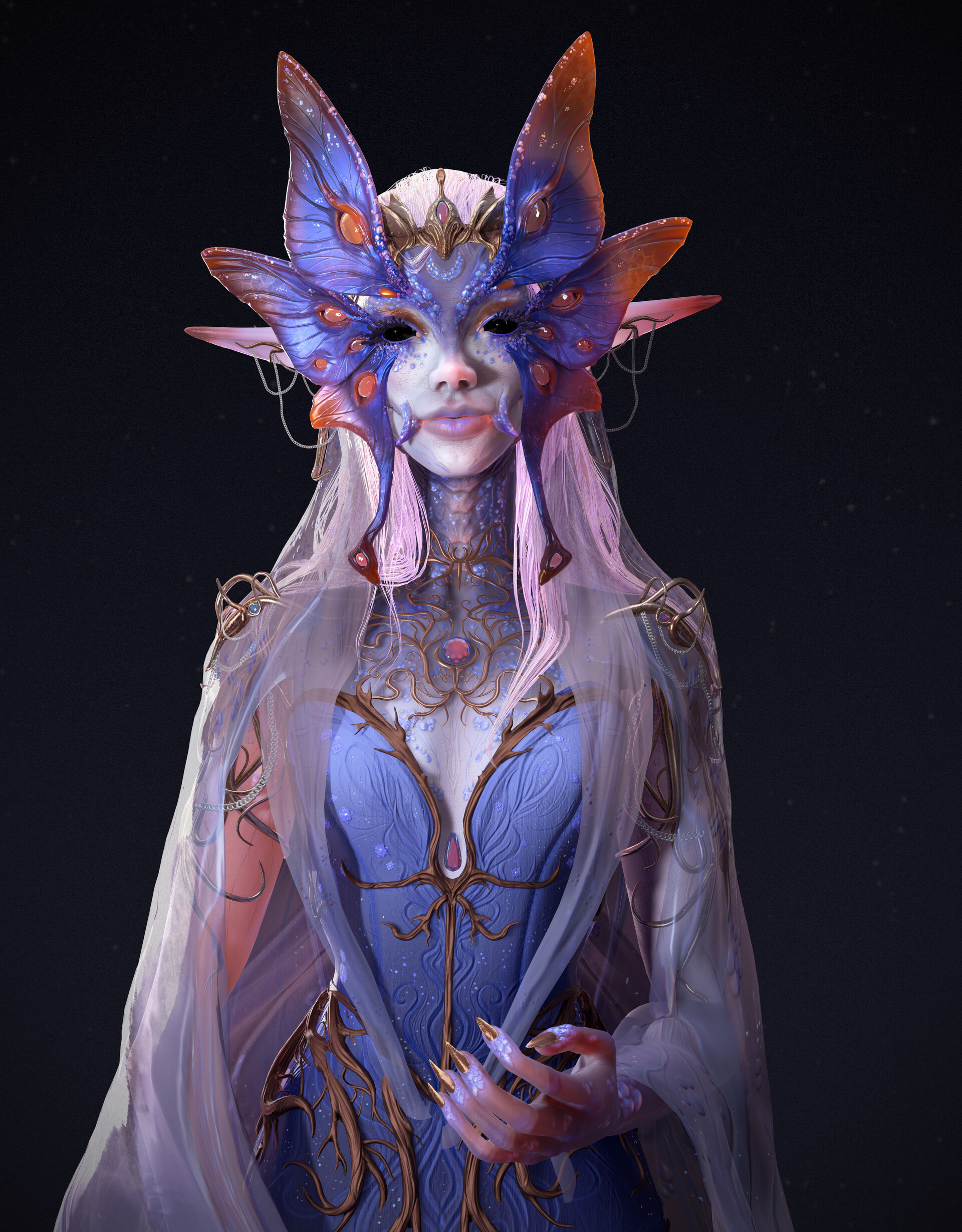This AI-generated image depicts a creepy and fantastical humanoid creature, blending human and surreal elements. The character, a woman with long whitish-pink hair, has a butterfly motif integrated into her facial structure, with butterfly wings emerging from the edges of her face. Unusually, these butterfly wings contain eyeballs, heightening the eerie effect. Her eyes, entirely black, lack the normal human features, enhancing the unsettling nature of her appearance.

She is adorned with a silver tiara and has ornate designs embellishing her skin, which is veiled by sheer fabric flowing from her head. Her attire includes a dark blue, intricately designed dress reminiscent of twigs and vines, complemented by a brooch at the neckline. The dress, with a purple bodice entwined with brown vines, extends to form a sheer cape. Her hands are a pinkish hue, sporting menacingly long, gold fingernail claws.

Overall, the image embraces a color palette of lilac purples and pinks, set against a completely black background, making the central figure vividly stand out. The fairy-tale-like character exudes an unsettling, surreal beauty, amplified by her elaborate jewelry and the fantastical, glittery butterfly wings crossing her face.